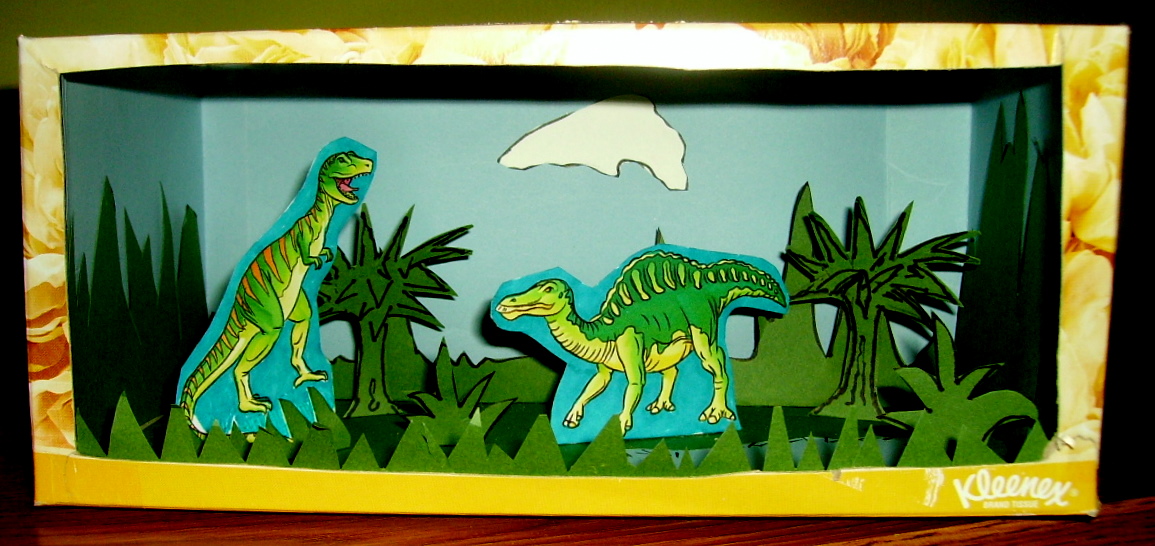This is a detailed color photograph of a Kleenex tissue box repurposed into a diorama, resembling a prehistoric scene potentially for a school project. The Kleenex box has a yellow and white marbled design and features the brand name "Kleenex" in the bottom right corner. The front and top of the box have been cut out to reveal a creatively crafted interior. The inside of the box has been painted blue to serve as the sky, with a single white paper cloud affixed at the back.

The diorama features two green dinosaur illustrations — a T-Rex standing on its hind legs with red stripes and another unidentified dinosaur on all fours with a yellow underbelly and yellow-green stripes on its back. Both dinosaurs face each other. Surrounding the dinosaurs are various illustrated cutouts of green trees and bushes, placed on both the left and right sides of the box as well as behind the dinosaurs, enhancing the prehistoric habitat feel. Along the bottom edge of the diorama, there are jagged pieces of what appears to be construction paper cut to resemble grass. The lighting in the photograph, possibly from a camera flash, highlights the gold-yellow hue of the box, adding a reflective shine.